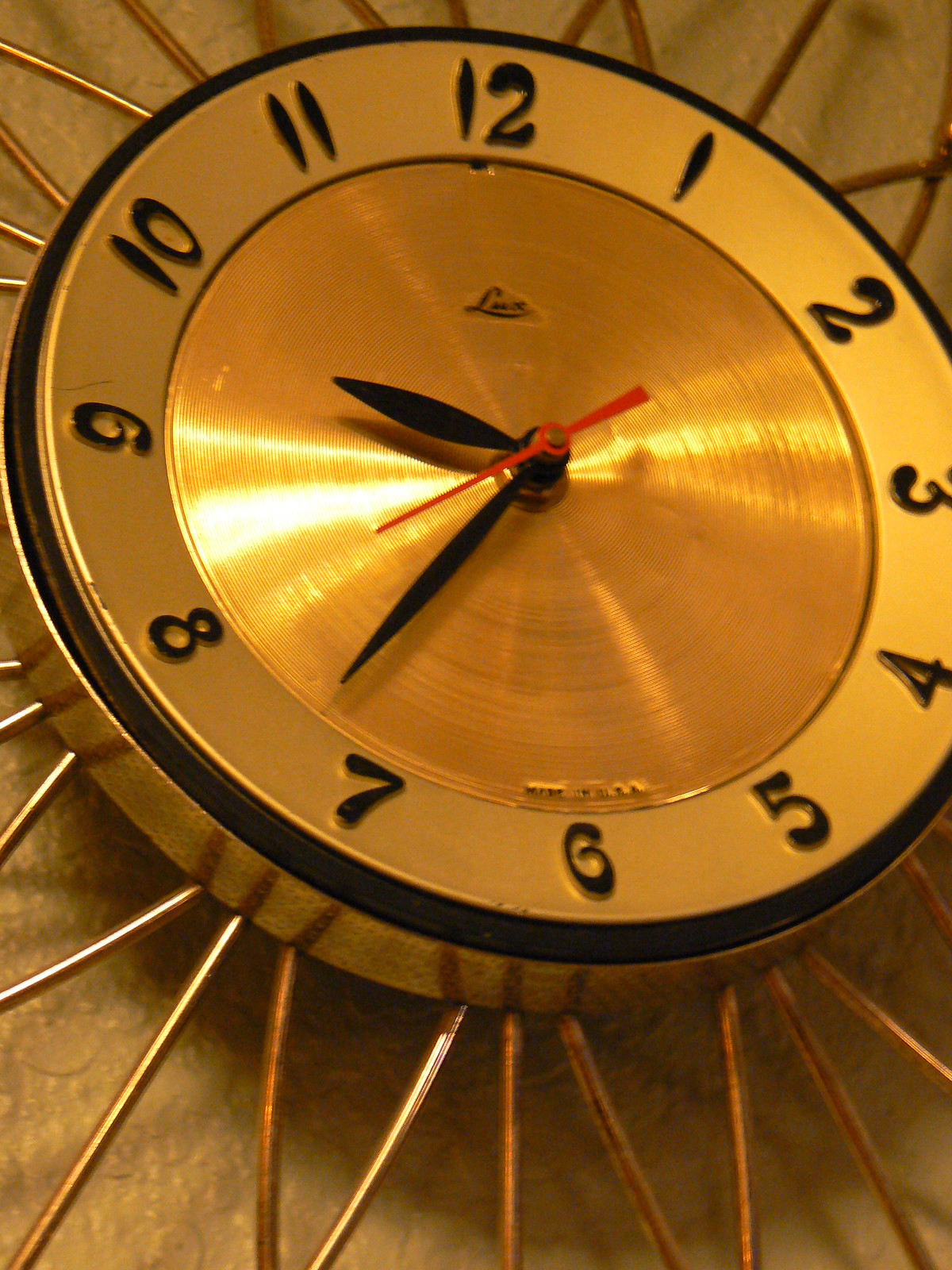This photograph features a striking, close-up view of a metal clock that dominates the entire frame. The clock, with its rich brassy hue tinged with brown, is encircled by a black trim. Each number, rendered in a somewhat whimsical, childlike font, is colored in bold black, standing out sharply against the backdrop. At the center, the clock showcases a section of brushed metal, adding texture and depth to the piece. The clock’s hands consist of a longer black minute hand, a shorter black hour hand, and a vibrant red second hand. Positioned just below the 12 o'clock mark, the manufacturer's name is faintly visible but remains illegible, while above the 6, the phrase "Made in the USA" is clearly embossed. Surrounding the clock are numerous metallic spikes in golden, silver, and copper hues, partially obscured but visibly intersecting and radiating outward from the clock’s rear, creating a dynamic and intricate pattern.